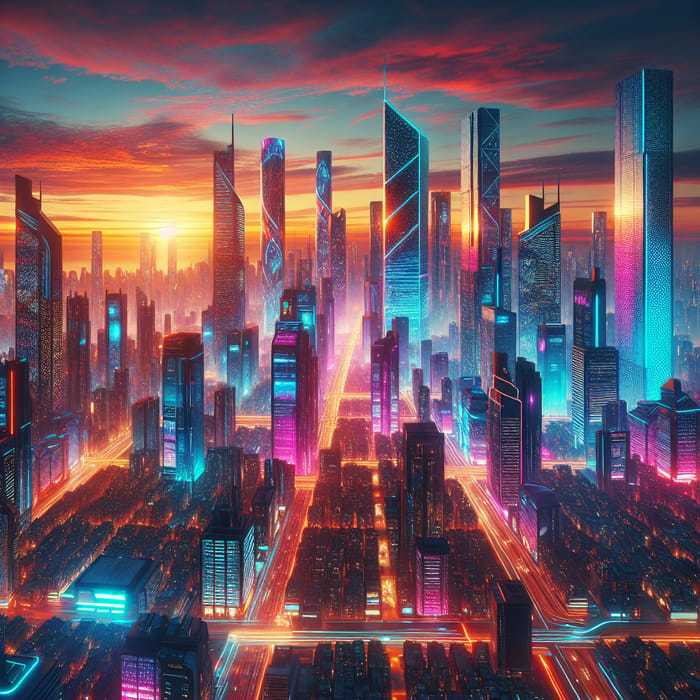This animated, computer-generated image depicts a futuristic city skyline at nightfall. The scene captures an array of skyscrapers, some towering between 50 and 100 floors, set against a dramatic sunset. The sun, positioned on the left horizon, bathes the sky in rich hues of yellow, pink, and red, which transition to dark blue at the topmost parts of the clouds. The city's buildings predominantly showcase shades of black and blue, with reflective surfaces that beautifully mirror the sunset's pink and yellow tones, giving them a neon glow. The city streets are illuminated in an unusual orange hue, likely a result of prolonged camera exposure, creating striking lines of light that resemble glowing wires snaking through the urban landscape. This cyberpunk vista is bathed in a surreal palette, blending natural and synthetic elements to create a visually arresting cityscape.